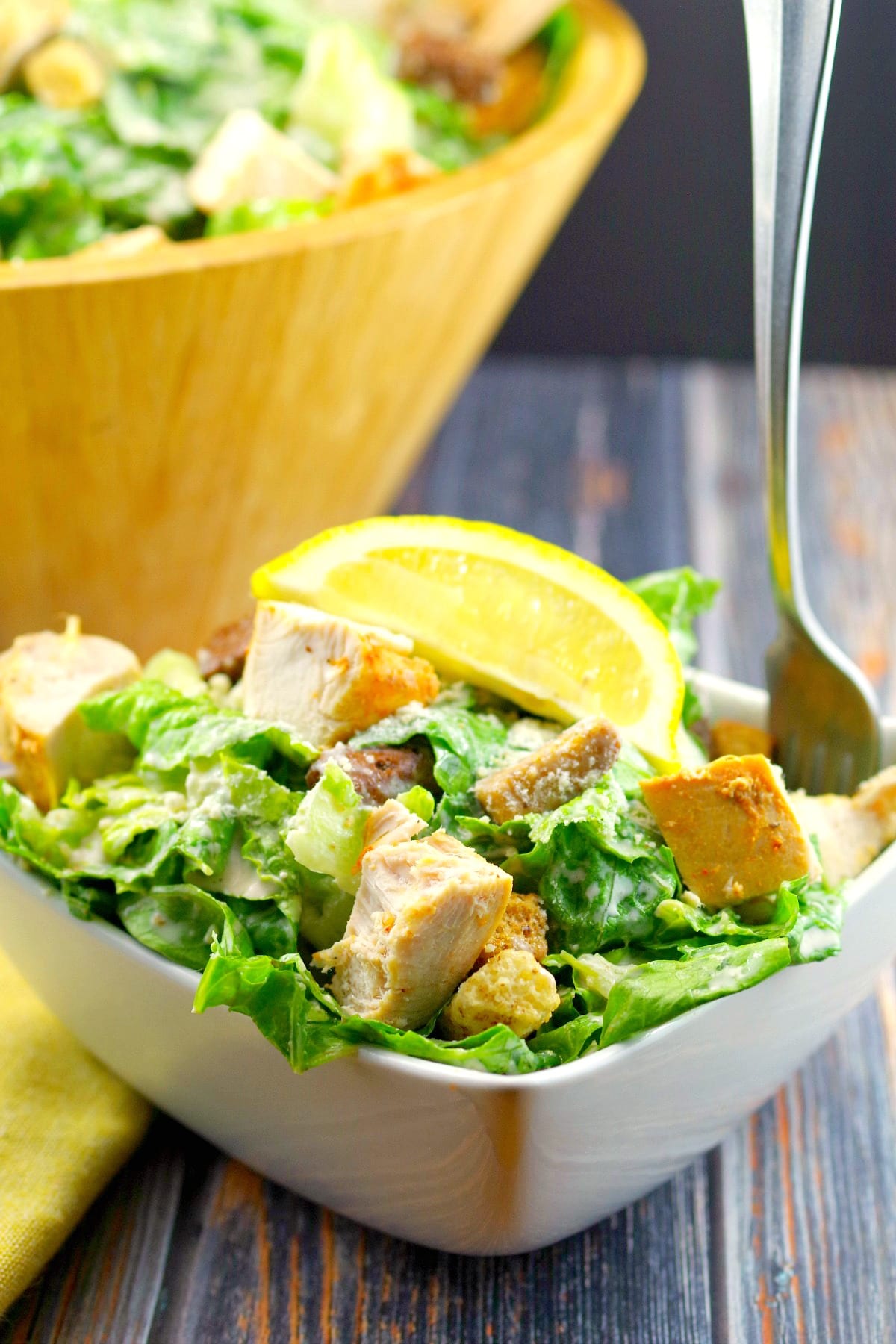This photograph features a detailed, close-up view of a small white ceramic bowl containing a chicken Caesar salad. The bowl, which is square in shape, sits prominently on a wooden plank table, accentuated by the presence of a yellow napkin to its left. The salad comprises vibrant green romaine lettuce, square chunks of light-tan chicken, crisp tan croutons, and a drizzle of white dressing. Topping off the salad is a bright yellow lemon wedge, positioned to add a fresh zest. Sticking vertically from the right corner of the bowl with its tines down into the salad is a fork, suggesting the dish is ready to be enjoyed. In the upper left-hand corner of the image, slightly blurred, is a larger wooden bowl containing more of the same salad, emphasizing that the portion in the smaller bowl is part of a larger serving. The overall focus of the image is on the small bowl of salad in the foreground, with no other background details present.